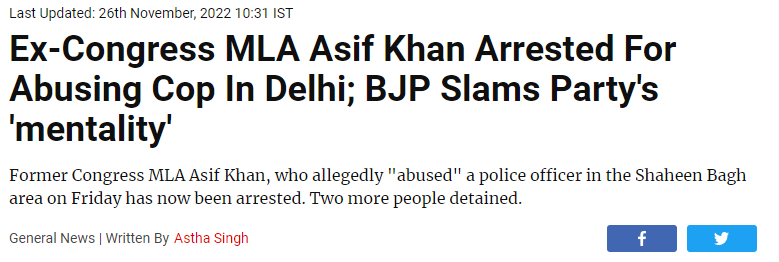Here is a cleaned-up and detailed caption for the image:

---

The image features a news bulletin with a white background. At the top, in a smaller black font, it reads, "Last updated: 26 November 2022 10:31 IST." Below this is a large, bold black heading that states, "Ex-Congress MLA Asif Khan Arrested for Abusing Cop in Delhi; BJP Slam Party Mentality."

The following paragraph, presented in standard black text, provides further details: "Former Congress MLA Asif Khan, who allegedly abused a police officer in the Shaheen Bagh area on Friday, has now been arrested. Two more people have been detained."

Underneath, in bold red text, the caption specifies the author's name: "General News written by Aista Singh."

On the right side of the image are two clickable social media icons: a blue rectangle with a lowercase white 'f' for Facebook and a lighter blue rectangle with a white bird for Twitter.

The rest of the image contains empty white space.